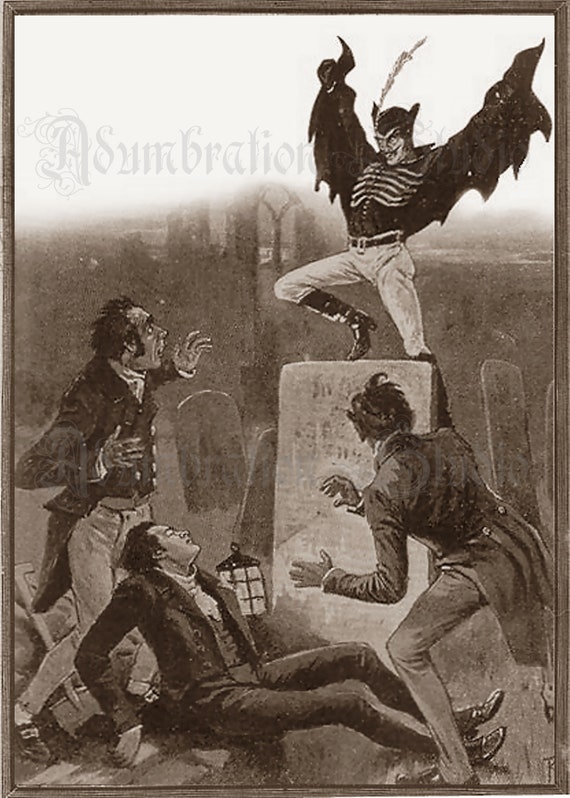The image appears to be an old, black-and-white illustration, likely from a book or possibly resembling a vintage movie poster. This vertically rectangular piece is framed by a gray border, with a faint caption at the top reading "A. Sombration" in light gray. Set in a cemetery at night and lit by a glowing lantern near a gravestone, the scene depicts a dramatic encounter. Standing atop the gravestone is a mysterious figure clad in light-colored pants, knee-high black boots, and a black shirt marked with a skeletal rib cage design. He wears a black cape, held aloft to resemble bat-like wings, and a partial mask revealing his face, giving him a vampiric or monstrous appearance. Below him, three men in long suit jackets react in terror. One man is sprawled on the ground, supporting himself with his hands next to the lantern, while the other two stand with their hands raised, eyes wide as they look up at the creature. The overall atmosphere is charged with fear and urgency, capturing a moment of imminent danger and supernatural suspense.